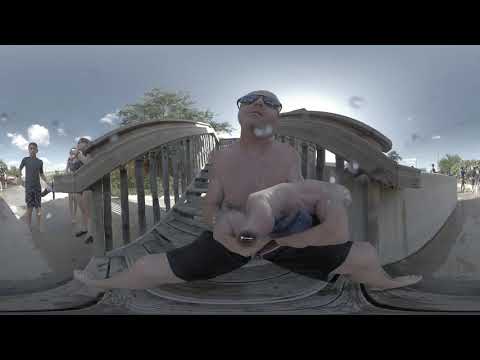In this fisheye-lens photograph, a shirtless man with fair skin and black swim trunks is seated on a wooden stairway, his legs splayed wide apart due to the distorted perspective. He appears to be holding an object, possibly a black selfie stick, with his hands extended in front of him. The man wears black swim goggles and sits upright, gazing upwards. Water droplets on the camera lens suggest a beach setting. The stairway features hand railings on both sides and is flanked by several people: three individuals, including a young boy and a woman, are visible to the left, while more people are scattered along a path to the right. The background includes a mix of trees and a partly cloudy sky with the sun peeking through, casting an unusual light on the scene.